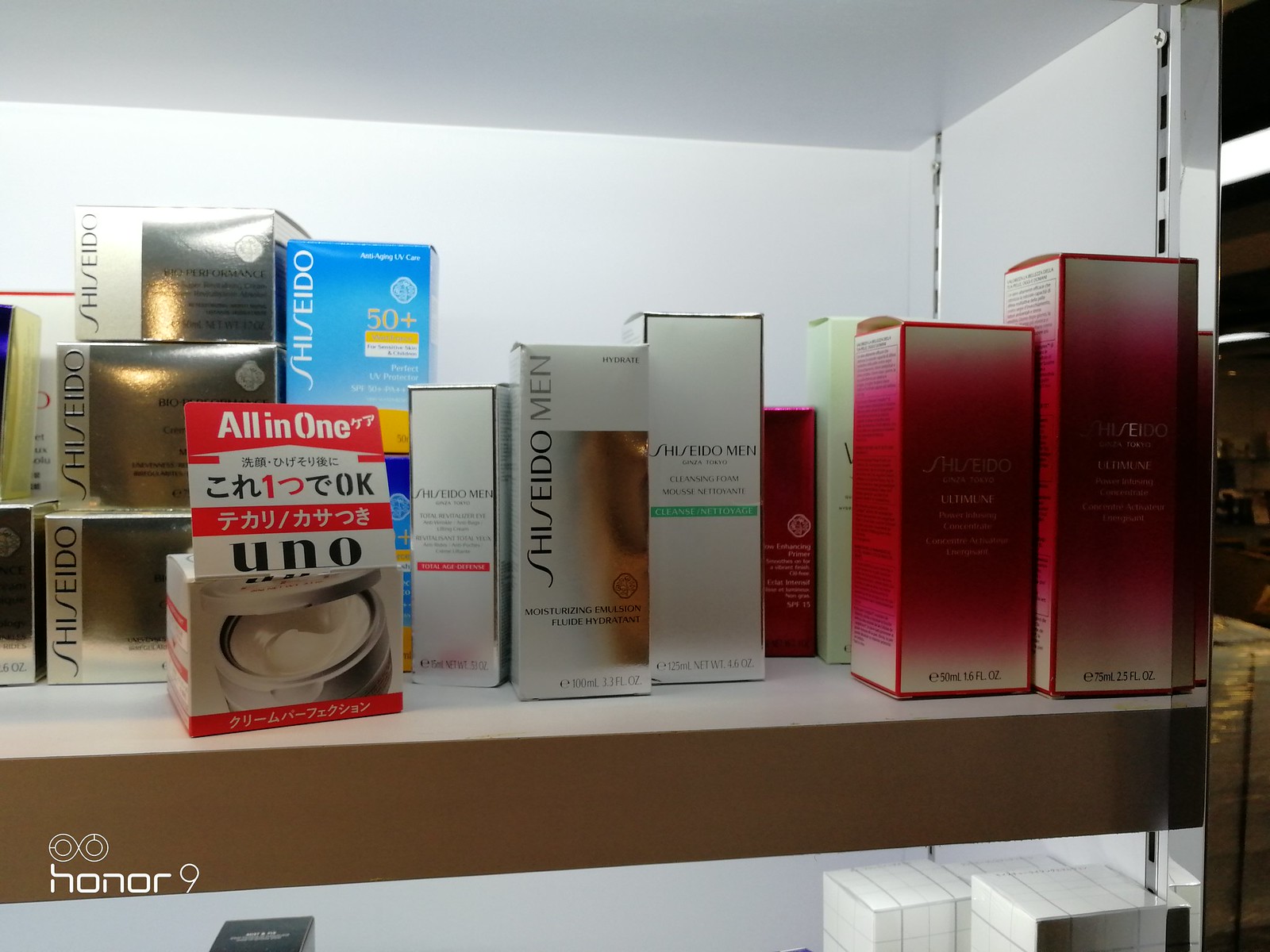A meticulously arranged shelf displays an array of boxed items, each varying in shape and size. Most boxes are distinct, with a few sharing similar characteristics. At the back of the shelf stands a prominent silver, square box labeled "Shiseido." Flanking this are several plain white or gray boxes, some also branded with "Shiseido," all approximately the same size. Towards the right, a colorful box with a pink and red gradient adds a vibrant contrast to the scene. In the lower left corner of the image, a transparent infinity symbol bears the inscription "Honor 9," adding an intriguing element to the composition.